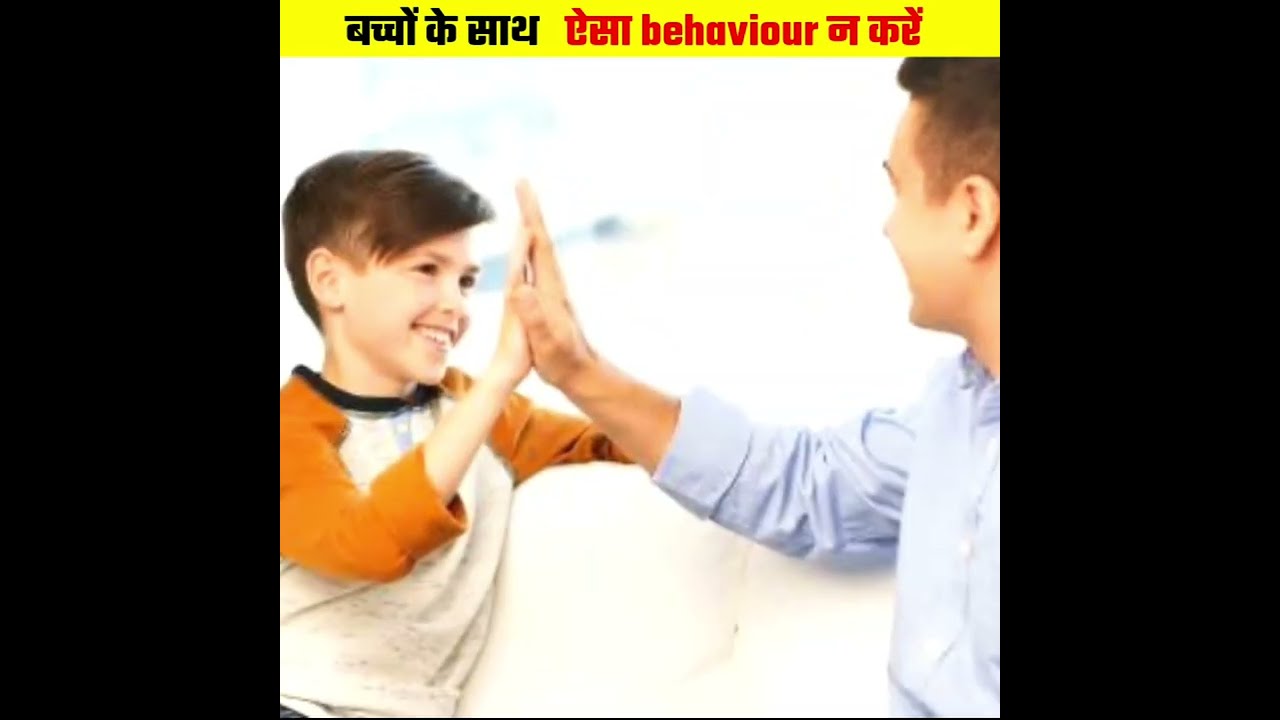In this photograph, a young boy and an adult man are sitting on a white sofa, joyfully giving each other a high five with their right hands. On the left sits the boy, wearing a white shirt with long orange sleeves and short brown hair swept to the side, and he is smiling directly at the man. On the right sits the man, dressed in a light blue long-sleeved shirt with the sleeve partially rolled up on his visible arm; he also has short brown hair and light skin. The background is washed out to a bright white, creating a clean and minimalist effect. The top of the image features a yellow horizontal strip with text, primarily in Hindi, that reads "बच्चों के साथ ऐसा behavior नहीं करें," with the word "behavior" written in English. Additionally, on the left and right sides of the image, there are black vertical strips that have a pearly, glitter-like appearance, adding a decorative touch to the borders.